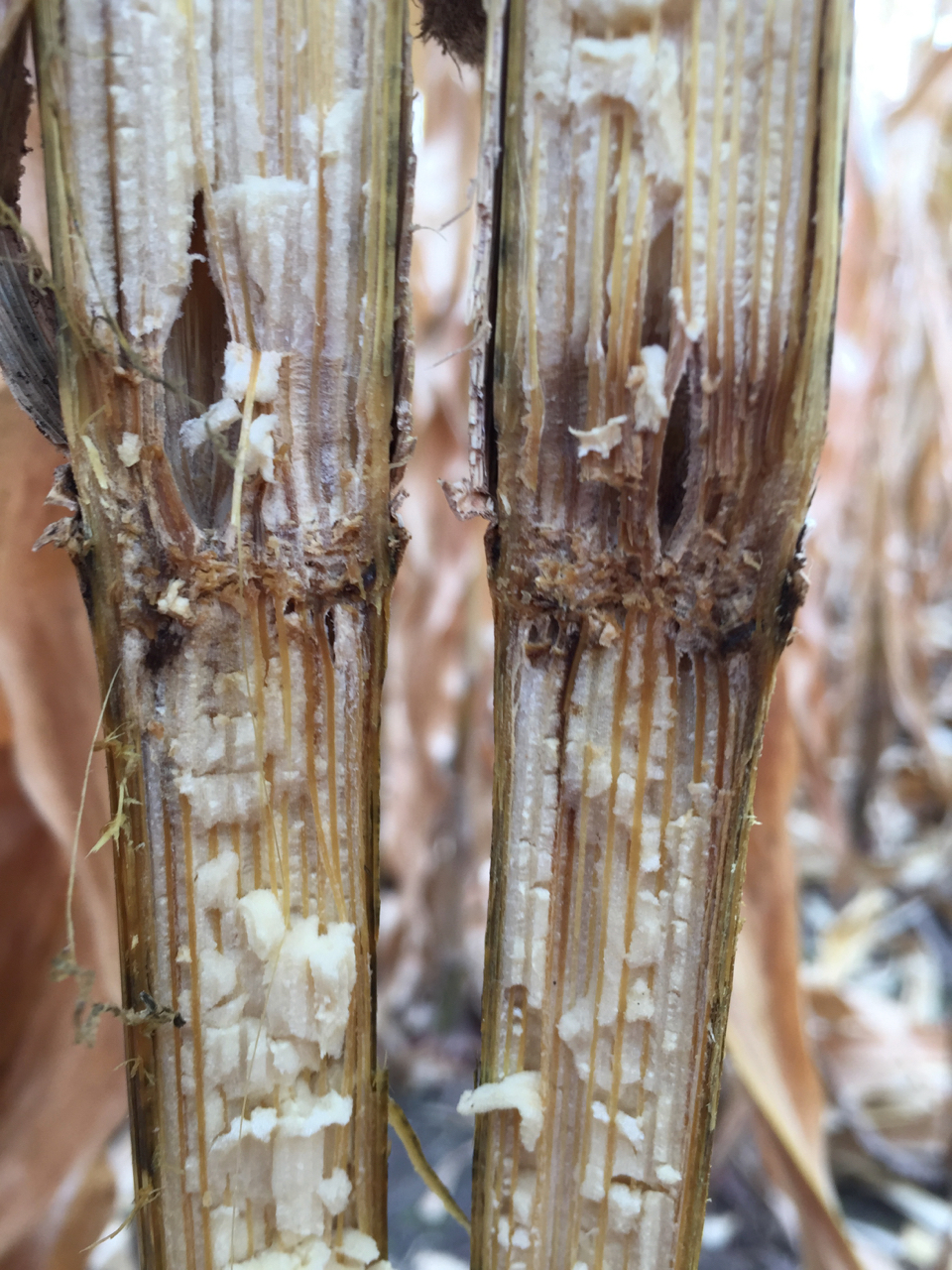This image is a close-up, highly detailed photograph of a plant stalk that has been cut in half, revealing its inner structure. The plant is beige with prominent white, fibrous material emerging from its core. The plant's interior on display is split into two parts, each showcasing vertical lines that could be vascular bundles or veins. These lines are a mix of yellow and green, numbering around seven in total. The white fibrous substance appears to be sloughing off and protruding between these lines. The background of the image is intentionally blurred, making it hard to distinguish specific details but presenting a blend of white, beige, and possibly hints of yellow and black, with an overall bright and focused appearance.